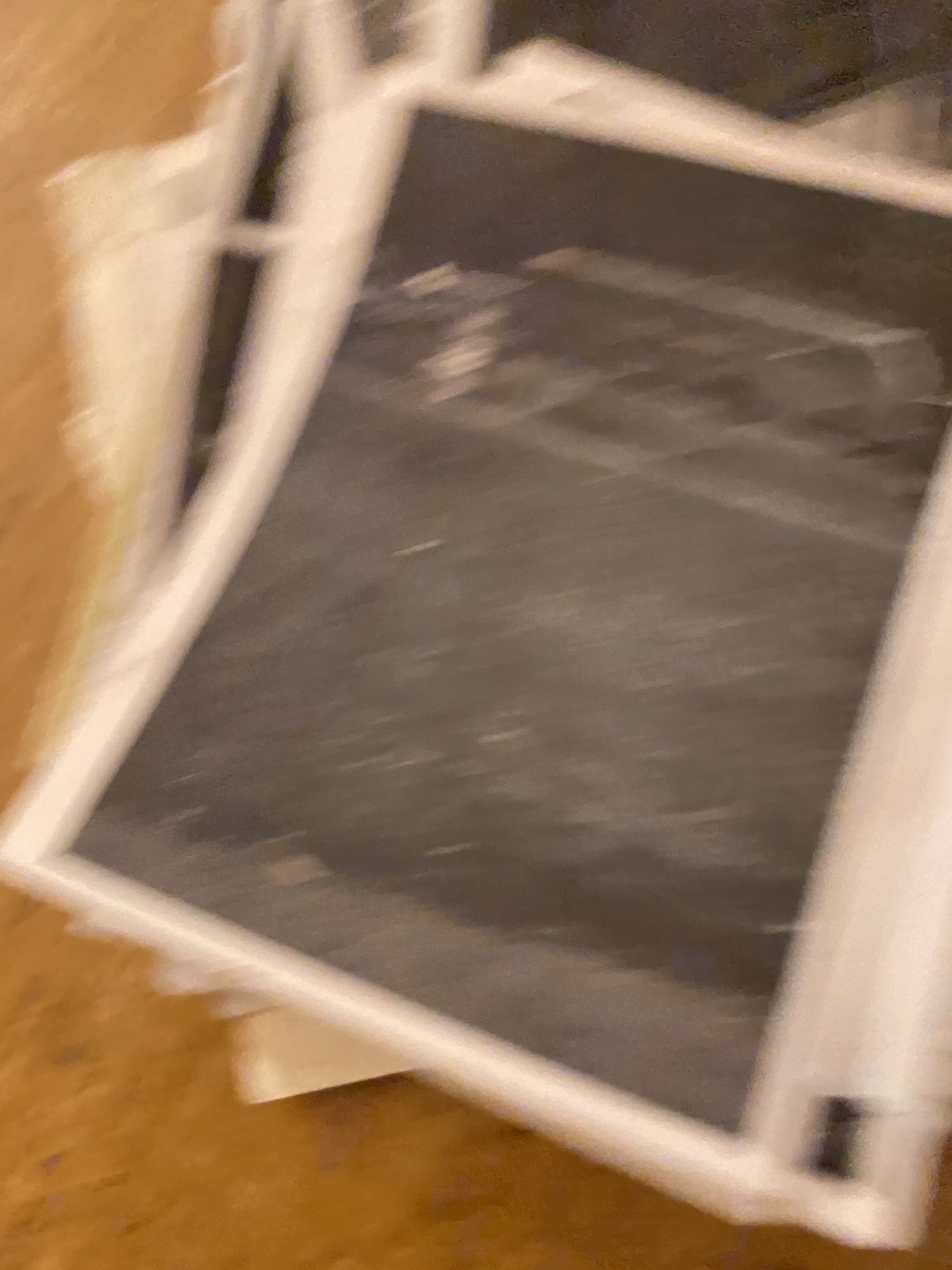The image depicts a highly blurred and indistinct scene, making identification challenging. The background appears to be a uniform brown, reminiscent of a dirt surface. Central to the image is an oblong object resembling a blackboard, similar to those used by children for drawing, though no markings or drawings are visible on it. This "chalkboard" is surrounded by a frame that is a mix of brown and white colors, not particularly vibrant but also not entirely dull. At the bottom of the framed object, there is a small black knob, which seems to suggest a feature for illuminating the drawing surface for better visibility.